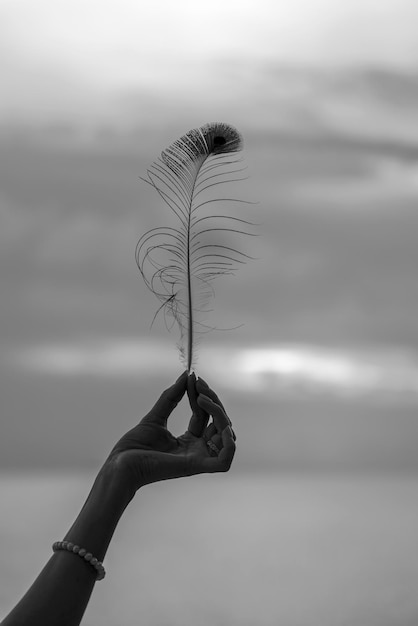This black and white photograph, vertically oriented, captures the delicate hands of a woman extending from the lower left corner of the frame. Her slender, styled fingers, with thumb and forefinger together, gracefully hold the very tip of a sparsely filled-out peacock feather, which reaches up to about a third of the way into the image. The feather appears to be blowing slightly in the wind, its strands not perfectly aligned. The woman is adorned with a string of pearls and a beaded bracelet halfway down her wrist. The background features a blurry, cloudy overcast sky and a suggestive gray plane that might be water, adding a serene, ethereal quality to the scene. This juxtaposition of intricate human detail and soft, natural elements underscores the delicate and fleeting beauty captured in this timeless moment.